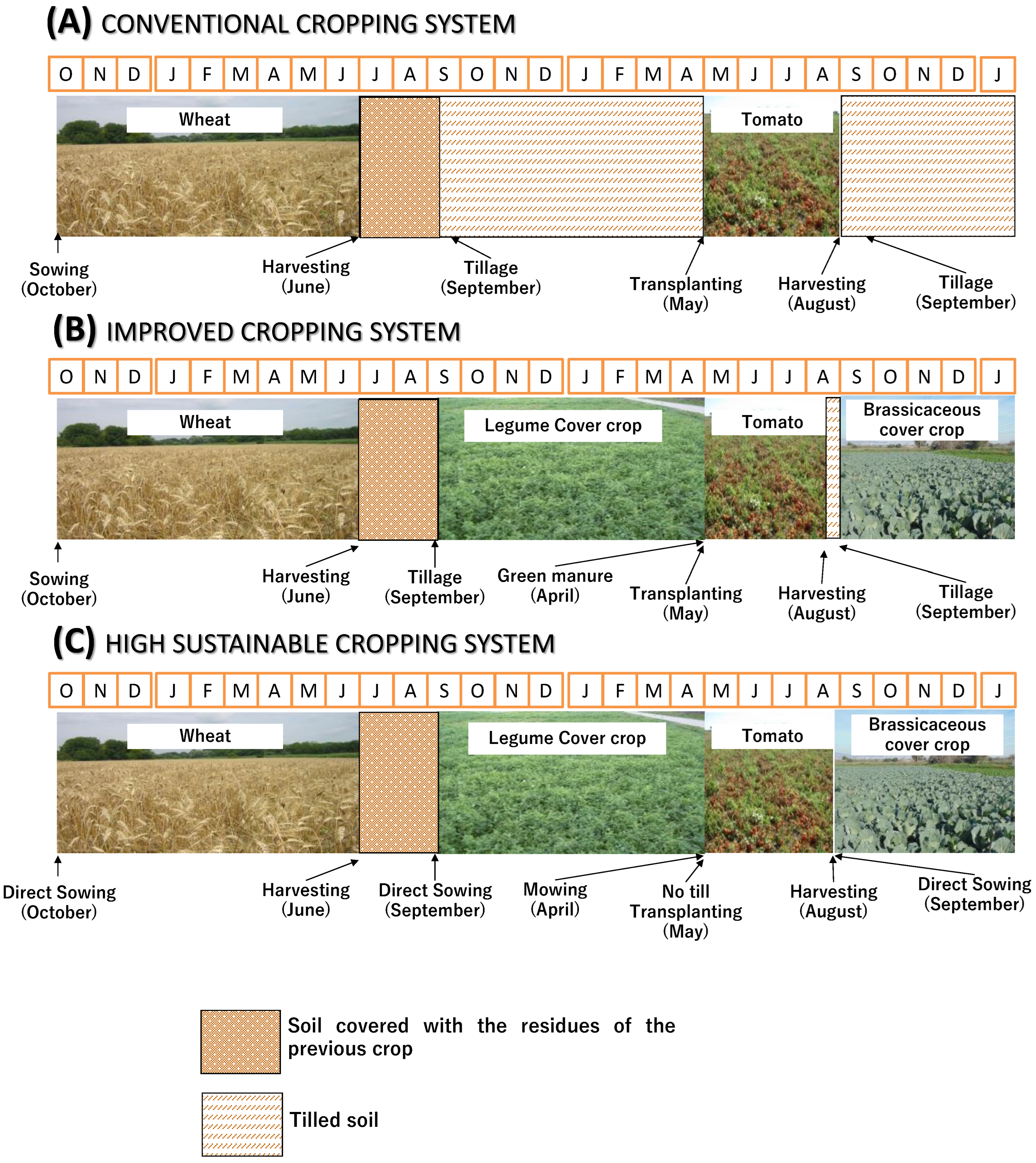The photograph depicts an infographic detailing three different cropping systems, labeled A, B, and C. 

- **A - Conventional Cropping System**: This section shows a sequence involving wheat and tomato cultivation. Wheat is sown in October and harvested in June, followed by tillage in September. Tomatoes are transplanted in May, harvested in August, and the soil is tilled again in September.

- **B - Improved Cropping System**: The improved system also starts with wheat sown in October and harvested in June, followed by tillage in September. In April, a legume cover crop is introduced as green manure. Tomatoes are transplanted in May and harvested in August. Finally, a brassica cover crop is used, and the soil is tilled again in September.

- **C - High Sustainable Cropping System**: This sustainable approach includes direct sowing of wheat in October, which is harvested in June, followed by direct sowing of a legume cover crop in September. The legume cover crop is mowed in April. Without tilling, tomatoes are transplanted in May and harvested in August. A brassica cover crop is also directly sown in September.

A legend at the bottom clarifies that orange indicates soil covered with the residues of the previous crop, while lines of orange signify tilled soil. The infographic spans various months from October to September and highlights the stages of sowing, harvesting, tillage, and transplanting in each cropping system.